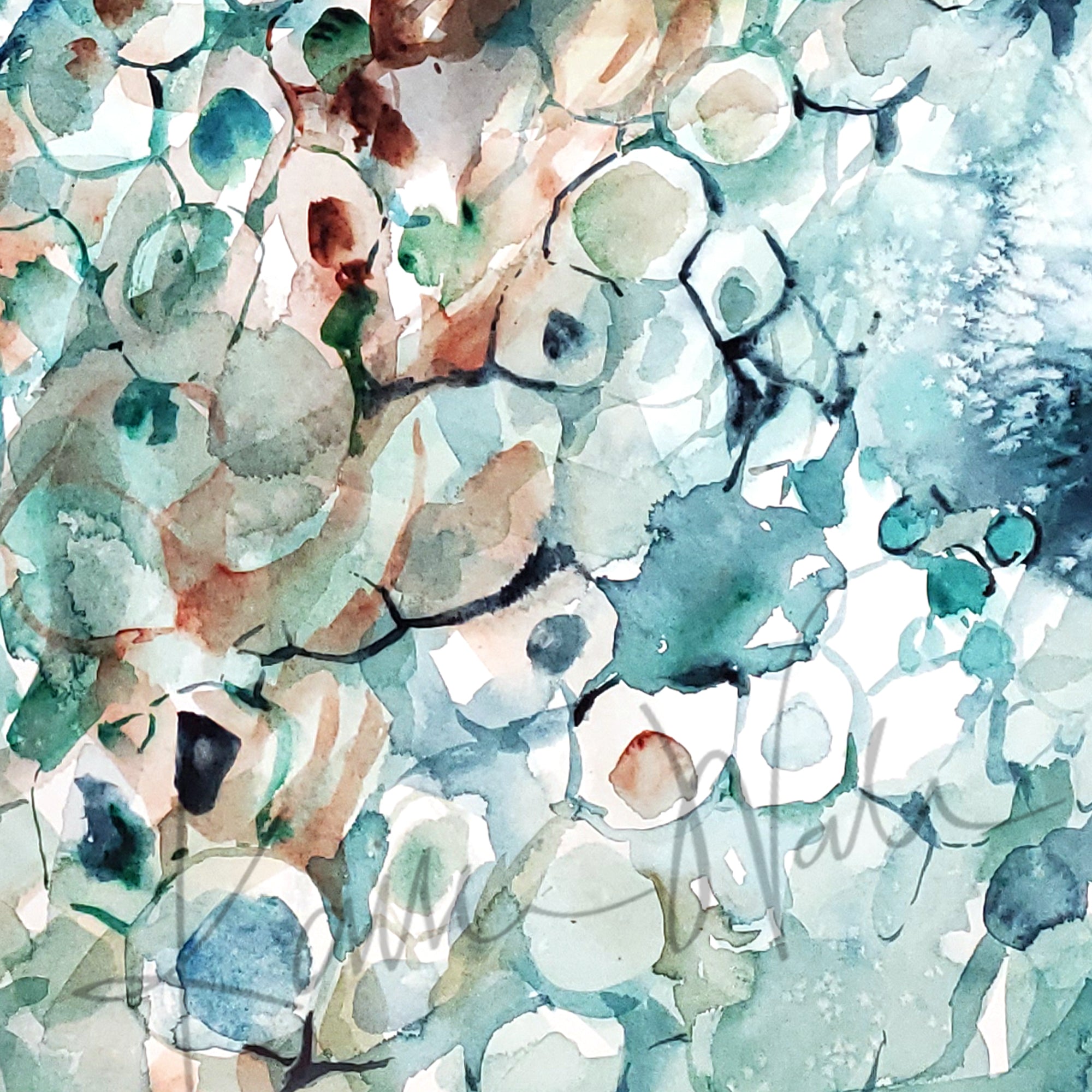The painting in the image is an abstract watercolor composition, approximately six inches by six inches in dimension. It prominently features a collection of colors, including blues, pinkish-tans, whites, grays, dark browns, and various shades of green. These colors form irregular, blot-like shapes that many observers interpret as flower-like forms. The painting has a sense of organized chaos, reminiscent of a microscopic view of cellular clusters, with these misshapen circles overlapping and densely packed, particularly on the left side of the image.

On the upper right corner, the scene transitions to a more fluid, blue-dominated area with small white elements that resemble a cloud of butterflies or shimmery highlights, adding a sense of movement and lightness. The darker reddish-brown hues are more concentrated in the top-left corner, gradually fading as they move towards the bottom-left. Scattered around the composition are multiple colors, giving an impression similar to a Van Gogh piece, where blooms and shapes are dispersed throughout the work.

Towards the bottom, spanning from left to right in a subtle light gray, the artist's signature is visible, though partially obscured and difficult to decipher. The name seems to be written as “Kantz-Nally,” though the exact spelling remains uncertain.